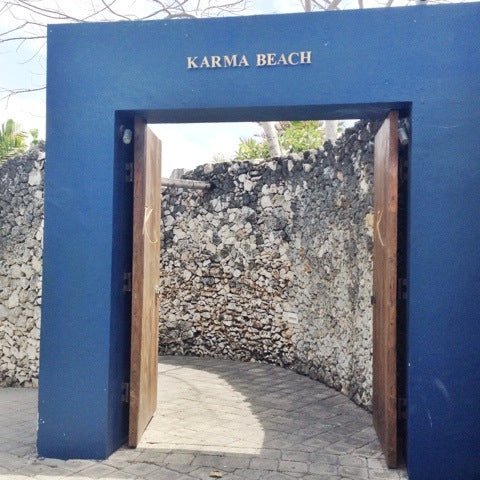This outdoor photo captures the entrance to an area called Karma Beach, highlighted by a bold blue entryway with a distinctive and eye-catching design. The entryway features two vertical blue pillars connected by a horizontal block at the top, where "KARMA BEACH" is displayed in prominent capital letters, likely gold or yellow in color. The structure frames two brown wooden doors, which are open, revealing a curving brick pathway. The bricks forming the path are small, square, and mostly brownish in hue. Flanking the path are tall walls constructed from an assortment of white, black, and gray stones. In the upper part of the image, you can see a glimpse of leafless tree branches, a stretch of blue sky, and white clouds, adding to the scenic outdoor ambiance. The overall impression is one of an elaborate, perhaps artistic, gateway reminiscent of the entrance to a high-end venue.